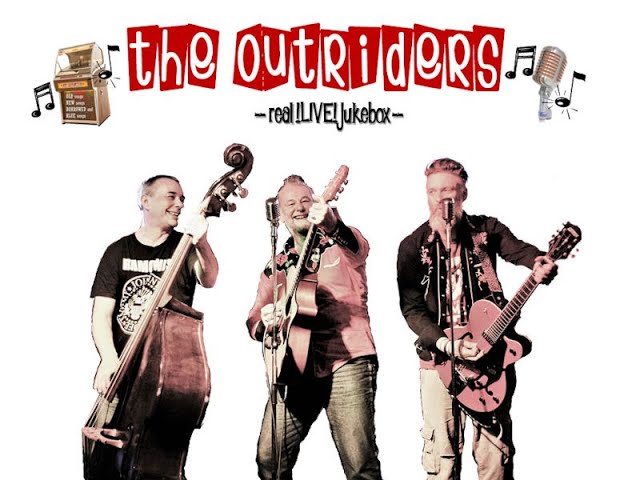The image in question is a poster or album cover for a music group named "The Outriders." The top of the poster features skewed red boxes, each containing a white letter, spelling out "The Outriders" in a bold, lowercase font. On the left side of the title, there's an illustration of a jukebox surrounded by musical notes, and on the right side, there's an old-style aluminum microphone with similar musical notes. Below the band's name, the black text reads "Real Live Jukebox," hinting at a rockabilly theme.

At the bottom of the image, the three band members are depicted. The man on the left wears a black t-shirt with white writing and plays an upright bass. He has short hair and smiles toward the center figure. The central figure appears to be the lead singer, dressed in a pinkish cowboy shirt with jeans, sporting puffed-up hair and also smiling. He plays an acoustic guitar and has a microphone in front of him. The man on the right, wearing a black cowboy shirt with pink designs and tan chinos, plays an electric guitar and has a microphone. All three men are older, potentially in their 50s, embodying a classic rockabilly style with their attire and instruments.